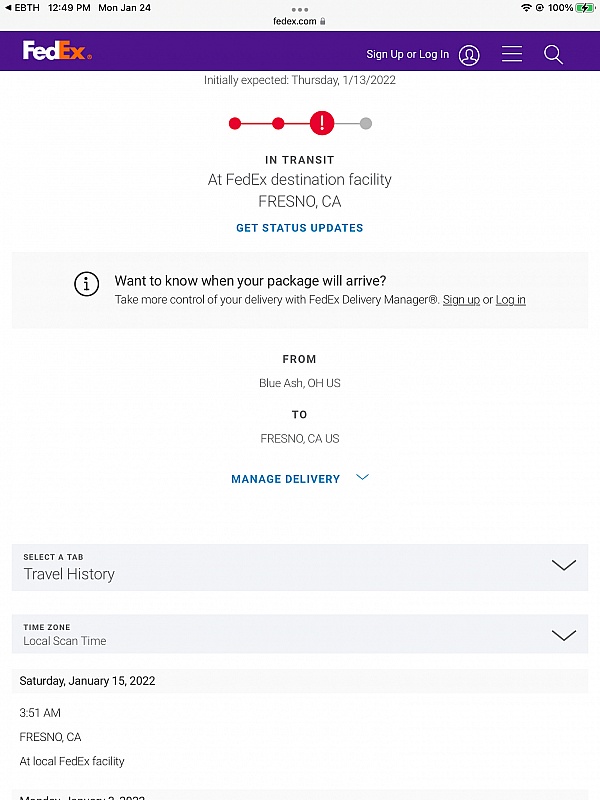The top right corner of the image shows a battery icon at 100% charge, marked with a small black lightning symbol. On the top left, the time is displayed as 12:49 PM, Monday, January 24th. Below this, a long purple rectangle features the FedEx logo on the left, with "Fed" in white and "Ex" in orange. Beneath the logo, text indicates that the package was initially expected on Thursday, January 13, 2022. Following this, a timeline with two small circles connected by a line leads to a larger third circle containing an exclamation point, signaling an alert or important status.

The next line reads, "In transit at FedEx destination facility Fresno, CA," in blue text, followed by a link for "Get Status Updates." Adjacent to this, an informational box with a lowercase "i" inside a circle prompts users with the message: "Want to know when your package will arrive? Take more control of your delivery with FedEx's Delivery Manager. Sign in or log in."

Below, the shipment's journey is detailed: from "Blue Ash, OH" (Ohio) in the U.S. to "Fresno, CA" (California) in the U.S. At the bottom, there is a blue option to "Manage Delivery."